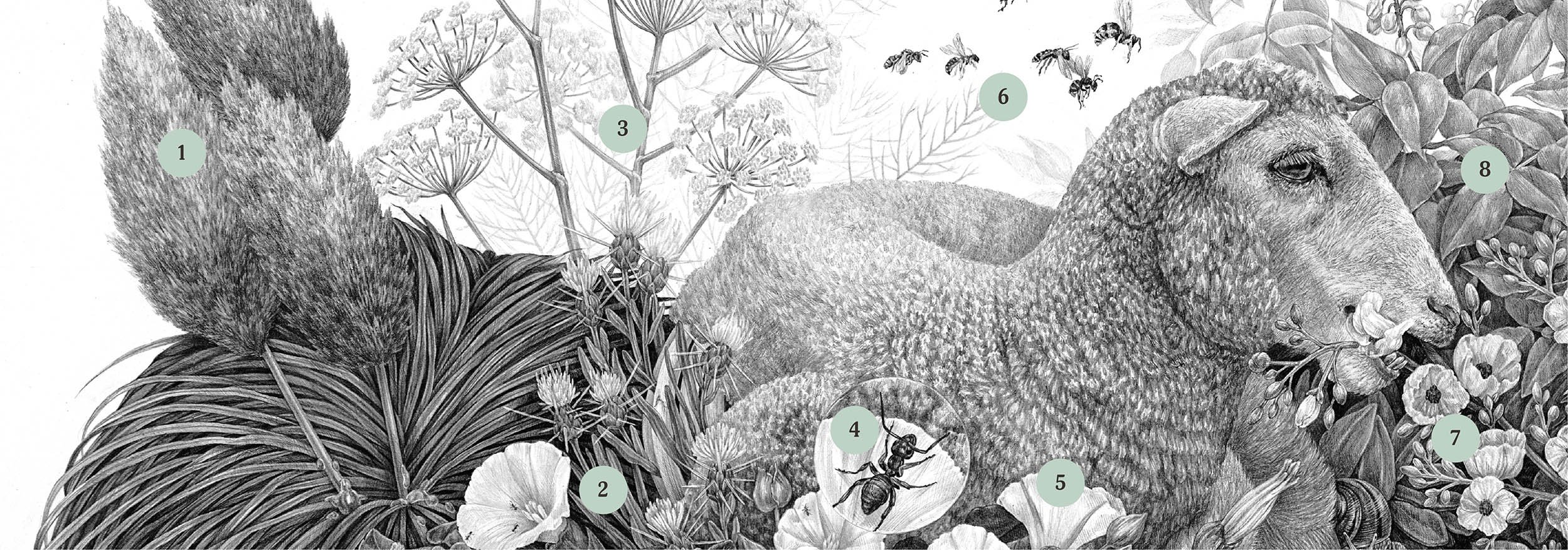In the black and white image, various elements of wildlife are meticulously detailed and numbered in dark green circles with black digits ranging from 1 to 8. The center of attention is a large mammal, distinctly appearing as a sheep with its coat trimmed short. Its eyes, ears, and open mouth are clearly visible as it seems to munch on a white petal flower, one of the few non-black-and-white elements in the drawing. Surrounding the sheep are diverse flora and fauna. 

On the far left, there is a plant with elongated leaves and next to it, a prominent white flower. Moving right, the third element is a different type of flower, resembling a dandelion. At position four, an ant is observed on a flower, seemingly magnified to show its detailed structure, and it appears to be near a droplet of water or dew. Further to the right, at position five, the sheep itself is documented. Buzzing around are several bees or winged insects. Continuing to the right, another distinct type of flower is marked at position seven, and finally, a cluster of leaves completes the scene on the far right.

The drawing, a sophisticated illustration possibly generated by a computer program, artistically captures a slice of nature with the sheep encircled by shrubs, flowers, and insects, blending the detailed elements harmoniously through varying shades of gray to nearly black tones, enriching the overall visual narrative.